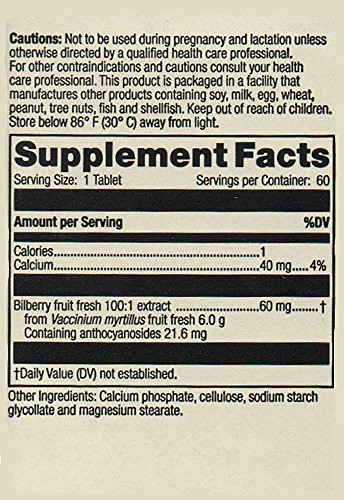The image is a portrait-oriented photograph displaying a nutrition label on a light background. The text on the label is printed in black, beginning with a bolded section that reads "Cautions:". Following this, in regular print, the label advises, "Not to be used during pregnancy and lactation unless otherwise directed by a qualified healthcare professional. For other contraindications and cautions, consult your healthcare professional."

The label also states, "This product is packaged in a facility that manufactures other products containing soy, milk, egg, wheat, peanut, tree nuts, fish, and shellfish." Additional safety instructions include "Keep out of reach of children. Store below 86 degrees Fahrenheit (30 degrees Celsius) away from light."

There is a bolded enclosed rectangle that highlights "Supplemental Facts," indicating the serving size of one tablet with 60 servings per container. The nutritional breakdown per serving lists:
- Calories: 1
- Calcium: 40 milligrams, constituting 4% of the daily value.

Further details specify that the product contains Bilberry fresh fruit 100:1 extract, with 60 milligrams derived from Vaccinium myrtillus fresh fruit (equivalent to 6 grams of fruit), providing 21.6 milligrams of anthocyanins.

The list of other ingredients includes calcium phosphate, cellulose, sodium starch glycolate, and magnesium stearate.